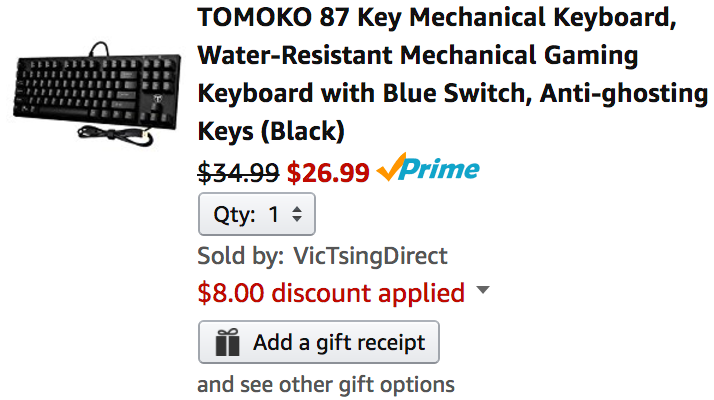This image is a cropped screenshot of a product listing on Amazon.com for a computer keyboard. On the left, there is a thumbnail image of the keyboard taken from an angled front view, facing left. The description to the right of the thumbnail reads, "Tomoko 87 Key Mechanical Keyboard, Water Resistant Mechanical Gaming Keyboard with Blue Switch, Anti-Ghosting Keys (Black)." The current price is prominently displayed in red as $26.99, reduced from the original price of $34.99, which is crossed out. The listing indicates the product is available for Prime shipping, featuring the recognizable Prime logo. Below the price section, a drop-down menu for selecting the quantity is set to 1. Further down, it notes the product is sold by a specified company and highlights an $8 discount applied in red text. There is also an option to add a gift receipt, with a prompt to "see other options" beneath that.